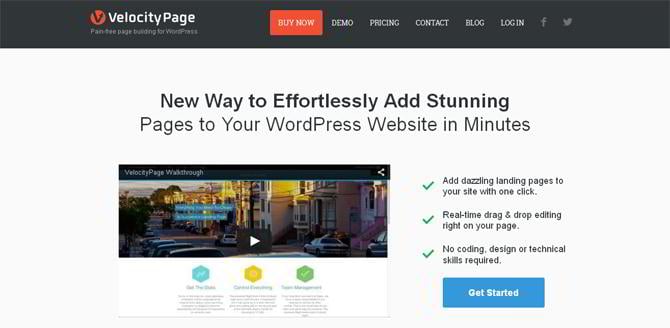**Velocity Page Website Screenshot: A Detailed Overview**

The top of the website showcases a sleek, black navigation bar with "Velocity Page" prominently displayed in white letters. Below the title, the tagline reads, "Pain-free page hosting for WordPress." Encapsulated in an eye-catching orange rectangle is a call-to-action button labeled "Buy Now,” along with navigation links for "Demo," "Pricing," "Contact," "Blog," and "Login." At the far right, icons for Facebook and Twitter are neatly aligned.

The main section of the page features a clean, white background with the headline, "A new way to effortlessly add stunning pages to your WordPress website in minutes." Dominating this section is a screenshot that appears to depict a picturesque city street reminiscent of San Francisco, complete with a variety of houses lining the left side and numerous cars parked along the road. While the text positioned underneath this image is too blurry to discern, the core message of the site is conveyed through a clear and concise checklist on the right:

- Add dazzling landing pages to your site with one click.
- Real-time drag-and-drop editing right on your page.
- No coding, design, or technical skills required.

This informative list is followed by a vibrant blue rectangle containing the text "Get Started" in white, designed to encourage immediate user engagement. 

The screenshot of the webpage is notably wider than it is tall, maintaining a streamlined and organized layout. Notably, there are no people, animals, or airplanes present in the image, allowing users to focus solely on the website's features and capabilities.